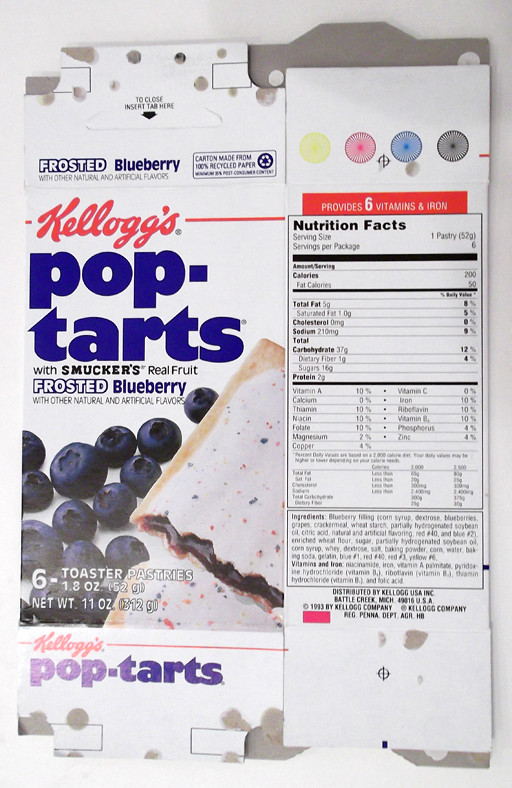This image features a flattened, empty box of Kellogg's Pop-Tarts with Smucker's frosted blueberry filling. The packaging prominently displays the brand name and product description: "Kellogg's Pop-Tarts with Smucker's Real Fruit Frosted Blueberry with Other Natural and Artificial Flavors." The front of the box is adorned with vibrant images of blueberries and a partially broken Pop-Tart, revealing the blueberry filling inside. The box indicates it contains six toaster pastries, each weighing 1.8 ounces (52 grams), with a total net weight of 11 ounces (312 grams), all detailed in white lettering.

The nutrition facts panel, set against a red background with white lettering, states that each serving size is one pastry (six servings per package). Each serving provides 200 calories, including 50 calories from fat. Key nutritional values include 5 grams of total fat (8% DV), 1 gram of saturated fat (5% DV), 0 milligrams of cholesterol, 210 milligrams of sodium (9% DV), 37 grams of total carbohydrates (12% DV), 1 gram of dietary fiber (4% DV), 16 grams of sugars, and 2 grams of protein. Additionally, the product contains 10% of the daily value for Vitamin A, thiamine, niacin, riboflavin, folic acid, and iron, among other vitamins and minerals.

The ingredients list includes blueberry filling (comprised of corn syrup, dextrose, blueberries, grape juice concentrate, and other components), enriched wheat flour, sugar, partially hydrogenated soybean oil, and various preservatives and colorings such as Red 40 and Blue 2. The product is distributed by Kellogg's.